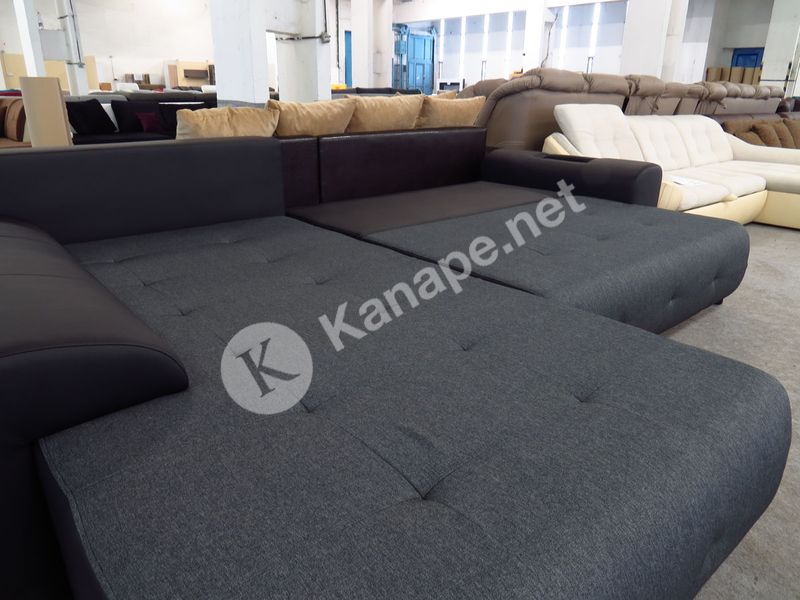This image depicts an indoor furniture showroom with a variety of couches and sofas arranged closely together. The backdrop features white walls interspersed with windows covered by blinds, allowing beams of sunlight to filter through. A distinctive blue door is visible in the background. In the foreground stands a prominent large, dark gray sectional couch with a lower armrest and high backrest. This sectional is adorned with a watermark, displaying a circular logo with a "K" and the URL "kanape.net," running diagonally from the lower left to the upper right. Surrounding the dark gray sectional, the showroom showcases other pieces, including white and taupe overstuffed sectionals, as well as various pillows. The furniture appears to be crafted from a mix of cloth and leather materials.